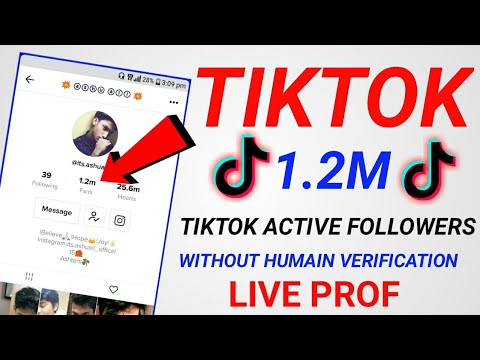A screenshot from a web page advertisement is captured in the photographic image. The image features black banners at both the top and bottom of the screenshot, while the central section is displayed against a clean, white background. Dominating the center is the TikTok name in large, bold red text. Accompanying it, in blue letters, is "1.2 million," clearly indicating a significant number.

Prominently displayed is the TikTok logo, resembling a music note in black, with a visually appealing green and red outline that creates a three-dimensional effect. Below the logo, the text "TikTok active followers" is printed in black, and its significance is further highlighted by the phrase "without human verification" in blue writing, which emphasizes the authenticity of the followers. Additionally, "live proof" is boldly declared in red text, enhancing the advertisement’s credibility.

The screenshot includes an image of a mobile device’s screen where a red arrow points conspicuously to the figure "1.2 million." The image also features an Indian male looking contemplatively to the side, with his hand by his mouth, giving a thoughtful impression. His follower statistics are shown: he is following 39 people and has garnered 25.6 million hearts on TikTok.